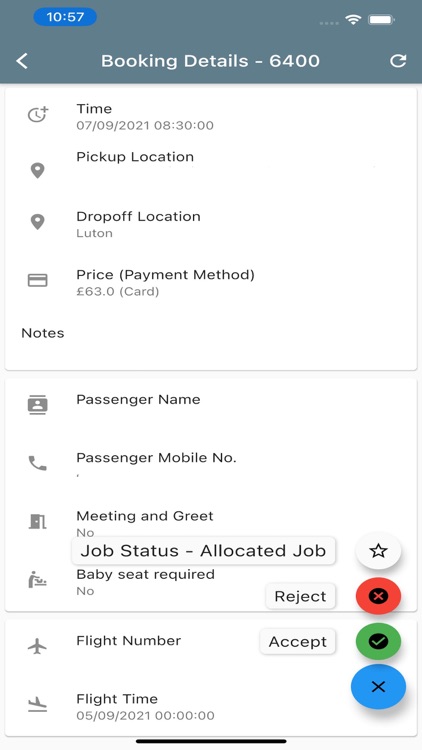This is a detailed screenshot from a mobile phone, showcasing a ride-hailing app interface, likely from Lyft or Uber. In the upper left-hand corner, the time reads 10:57. Dominating the top of the screen is a dark gray bar featuring the text "Booking Details - 6400" in one of the largest fonts visible. The booking time is noted as 8:30 on July 9th, 2021. Below this, the interface lists both the pickup location and the drop-off location, which in this case is Luton. 

Further down, the price and payment method are displayed, indicating that the currency is in pounds, confirming that the location is within the UK. 

In the lower right-hand corner, there are four notable circles, each with distinct icons: the top circle contains a star, the second one from the top has a red X, the third one down shows a green checkmark, and the bottom circle is marked with a blue X, likely the app's close button. Moreover, fields for notes, the passenger's name, and the passenger’s mobile phone number are visible, organizing all needed details for the ride.